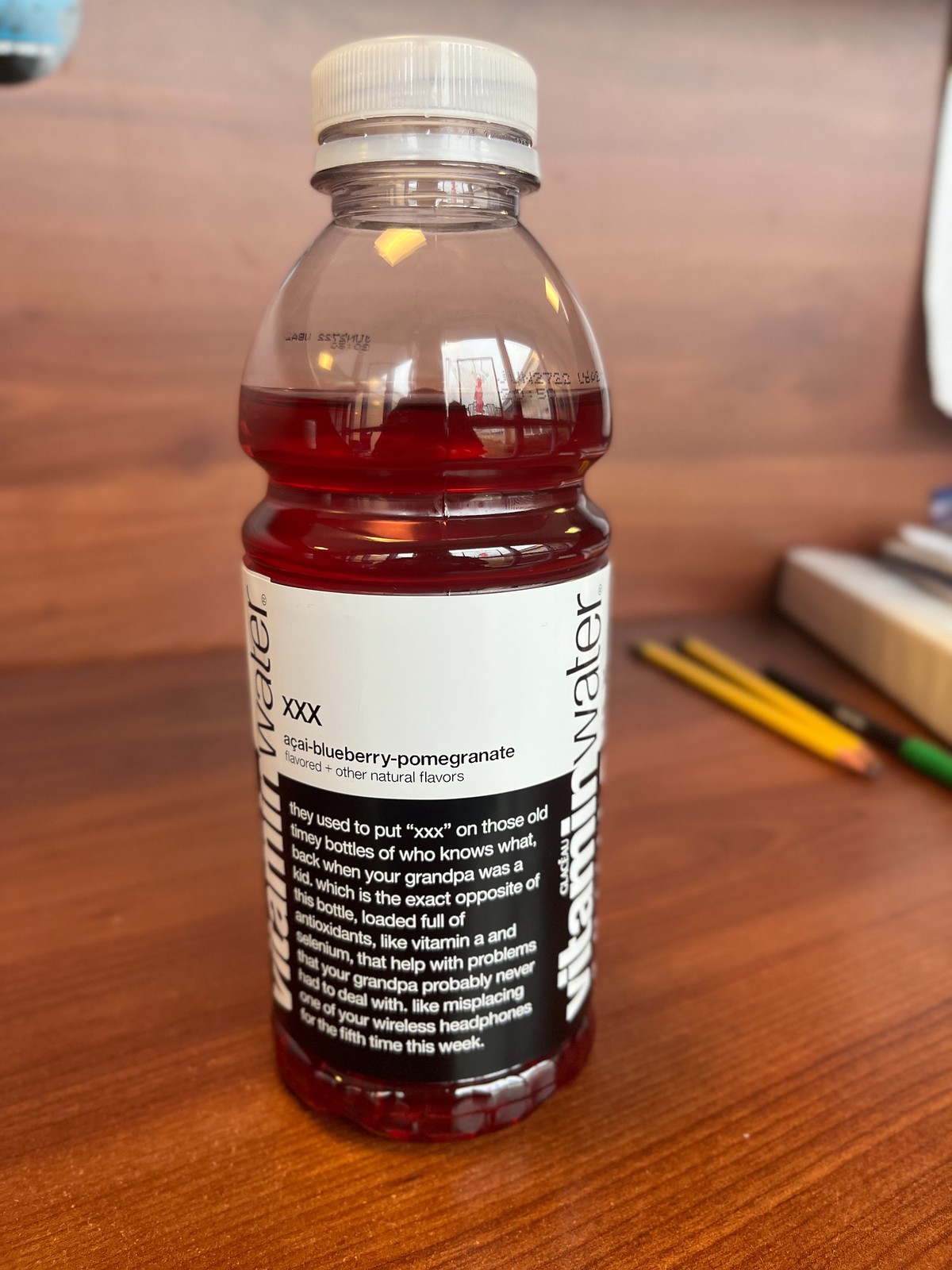The image showcases a side view of a bottle of Vitamin Water placed on a richly colored, medium-brown wooden table. The bottle contains a red liquid and features a white label with black and white text. The label prominently displays "Vitamin Water" written vertically. The visible part of the label indicates the flavor as "Blueberry Pomegranate" in black text. Below this, there is a black section with white text, which includes a nostalgic message about how they used to put "XXX" on small bottles of an unknown substance back in the days of one's grandfather, although this text fades and is partially illegible. To the right of the bottle, there are two yellow pencils alongside a black and green pen.